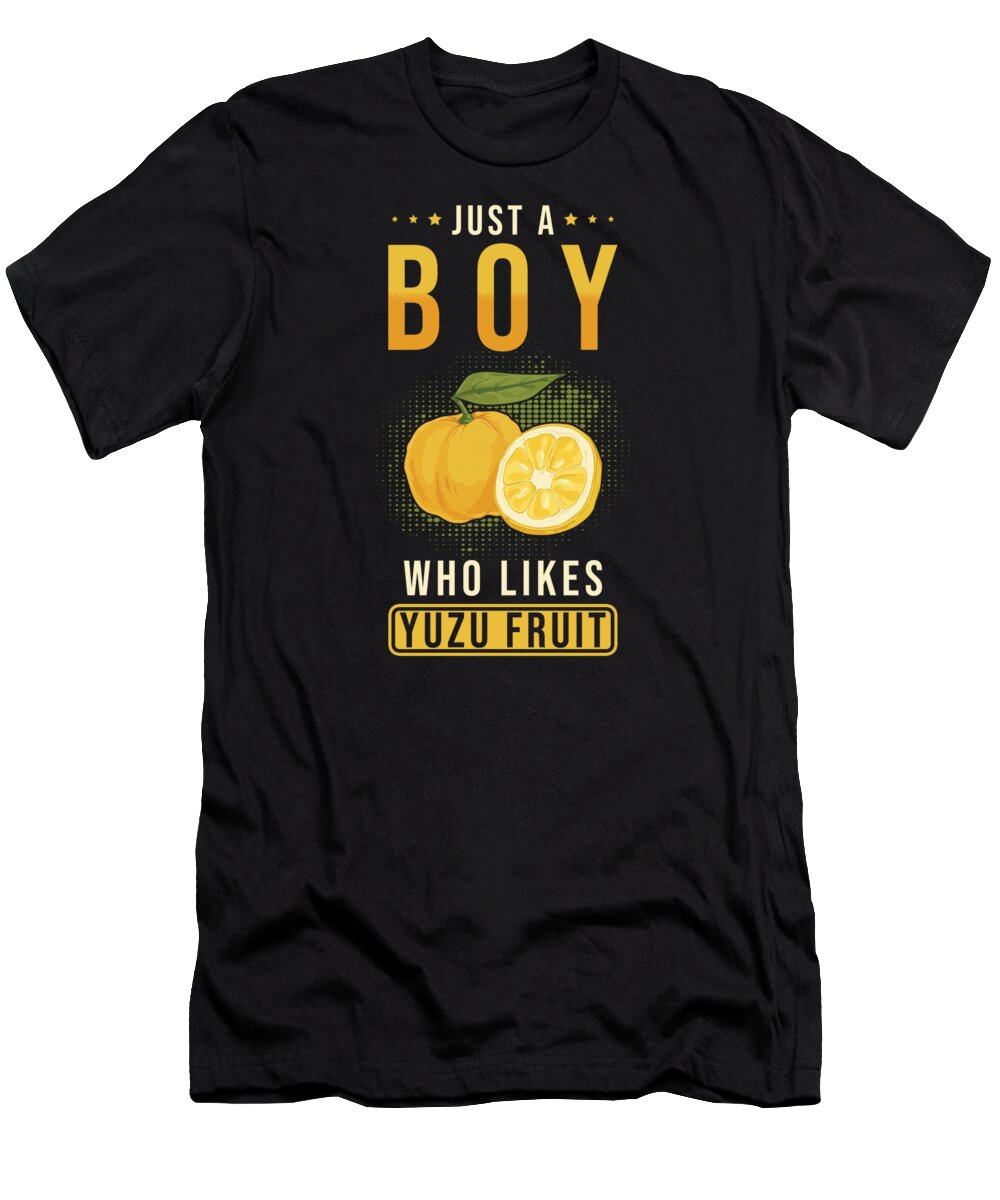The image showcases a slightly wrinkled black t-shirt against a white background. Centered at the top, in white font and flanked by three progressively larger golden stars on each side, is the text "just a." Below this, the word "boy" is prominently displayed in a larger yellow gradient font, transitioning from orange at the bottom to yellow at the top. Midway down the shirt is a vibrant depiction of a whole yellow lemon on the left and a sliced lemon on the right, embellished with a pixelated grid background and a green leaf. Underneath the lemon graphic, the phrase "who likes" is written in smaller white font. Finally, at the bottom, in a yellow rectangular box with black font, the words "yuzu fruit" are displayed. This detailed design is positioned towards the top center of the t-shirt.